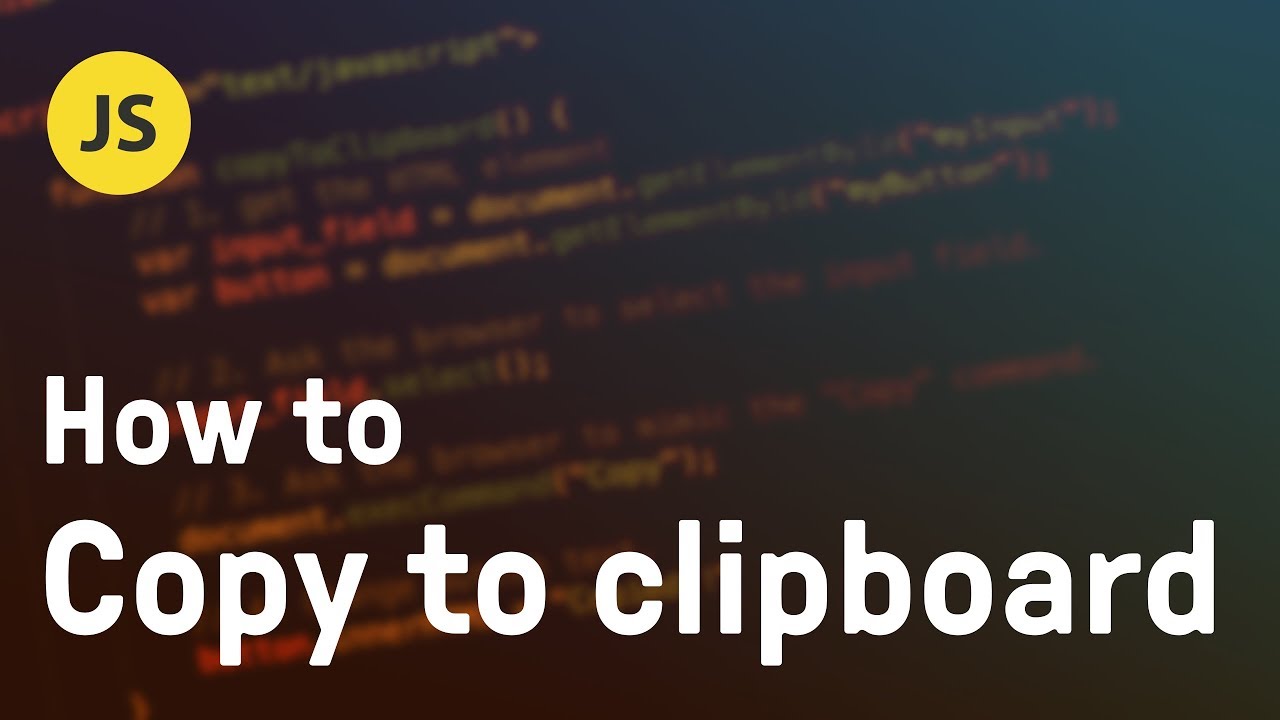The image features a screenshot with a blurred background containing a mix of red, yellow, green, and black coding elements. In the upper left-hand corner, there's a distinct yellow circle with the black text "JS" written in capital letters. At the bottom of the image, a thick, medium-sized font spells out "How to Copy to Clipboard" with specific capitalization: the 'H' in 'How' and the 'C' in 'Copy' are capitalized, while the 't' in 'to' and the 'clipboard' are in lowercase. The coding in the background, although blurred, exhibits a colorful mix of red, yellow, and green against a predominantly black, faded, and cloudy backdrop.